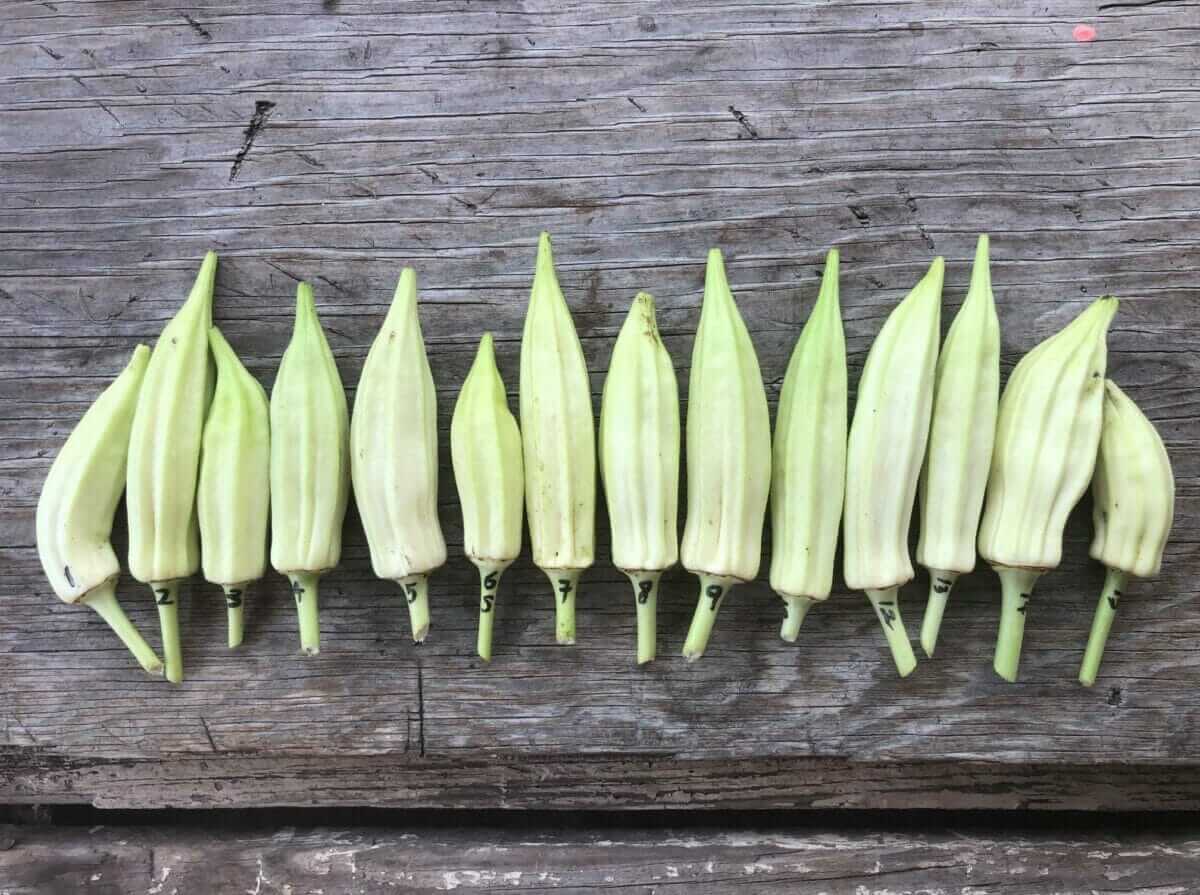This photograph features a row of 14 yellowish-green, pepper-like fruits, possibly a unique variety of peppers, each with distinct vertical ridges. They are meticulously laid out in a horizontal line across weathered gray and brown wooden boards, contributing to a rustic aesthetic. The fruits range in shapes and sizes, with some being long and slender while others are shorter and more squat. Each fruit is marked with a black number, starting with 1 on the left and progressing irregularly through 14 on the right, though some numbers appear to be missing or obscured. The stems, located at the bottom of the fruits, give them a slight resemblance to bananas.